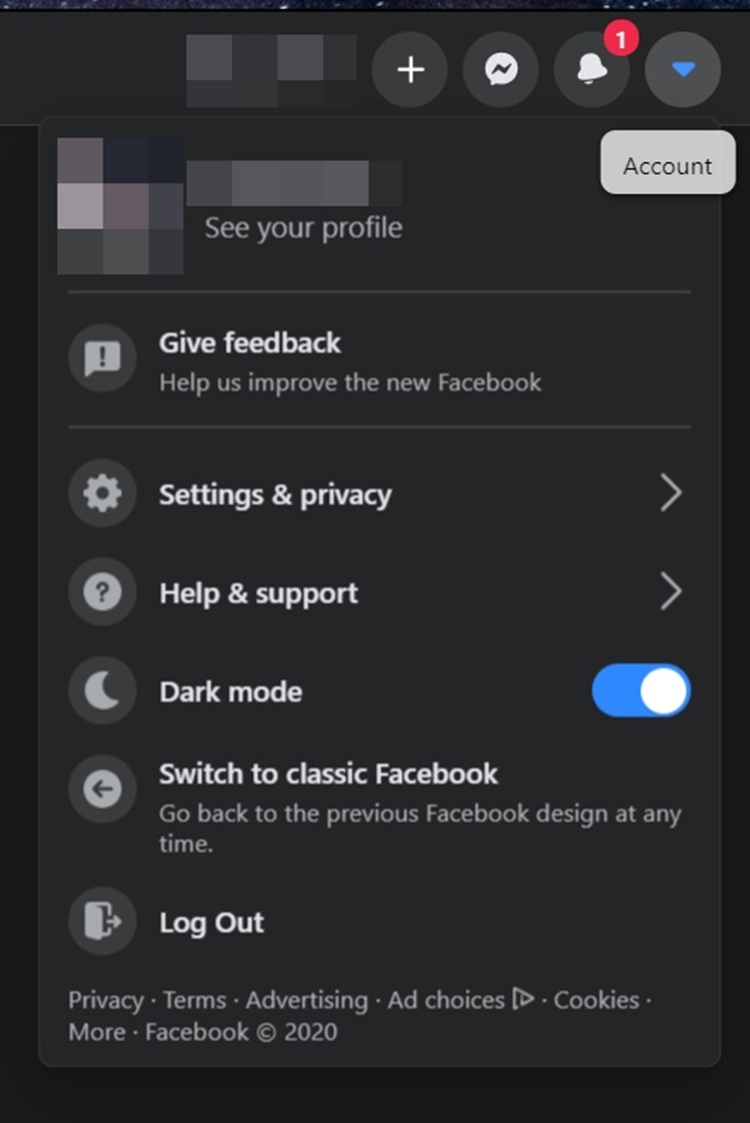A detailed view of an app interface is displayed. The main layout is a vertical rectangle resembling the shape of a typical phone or tablet screen.

At the top-right corner, there are four distinct icons:
1. A plus symbol.
2. A white circle with the letter "N" inside.
3. A white bell icon with a red circle and a numeral "1" inside, indicating an alert or notification.
4. A blue triangle with a box underneath labeled "Account."

On the left side of the top section, there are several blurred-out squares, possibly concealing additional elements, perhaps about a dozen in total.

Below these icons, there is a profile section which likely includes the user's name and profile photo. Following this are key options arranged vertically down the center:
- Give Feedback
- Set to Privacy
- Help and Support
- Dark Mode (indicated as activated with a blue toggle button on the right)
- Switch to Classic Facebook
- Log Out

All these options are displayed in blue font, with corresponding icons either on the right or left side of the text.

At the bottom of the screen, standard links for Privacy Terms, Advertising, and other informational links are provided. The footer note "Facebook 2020" confirms that this interface belongs to the Facebook app.